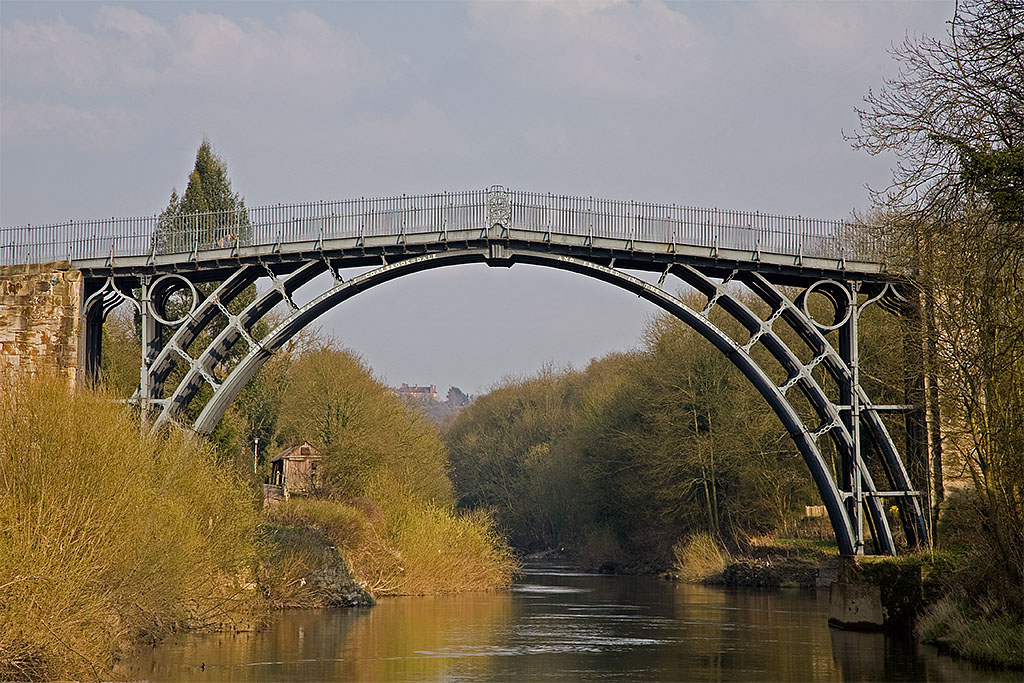This detailed photograph captures a serene scene of a silver metal bridge arching gracefully over a calm waterway or river, with decorative circular and horizontal elements adorning its structure. The bridge, which appears to be a pedestrian walkway, features protective metal railings and is slightly elevated, flanked by stone pylons at both ends. The landscape on either side displays rocks cemented together, lush green bushes, reedy grassy plants, and trees—one notably tall and green—alongside the riverbanks. A weathered brown wooden building with an exterior light can be seen on the left-hand side near the bridge, contrasting with the much broader cityscape visible in the far distance. The overall lighting of the scene is characterized by a gray-blue hue, complemented by a backdrop of a dark blue sky interspersed with wispy white clouds. This setting, encased in winter foliage with bare branches, conveys a peaceful, almost timeless essence.